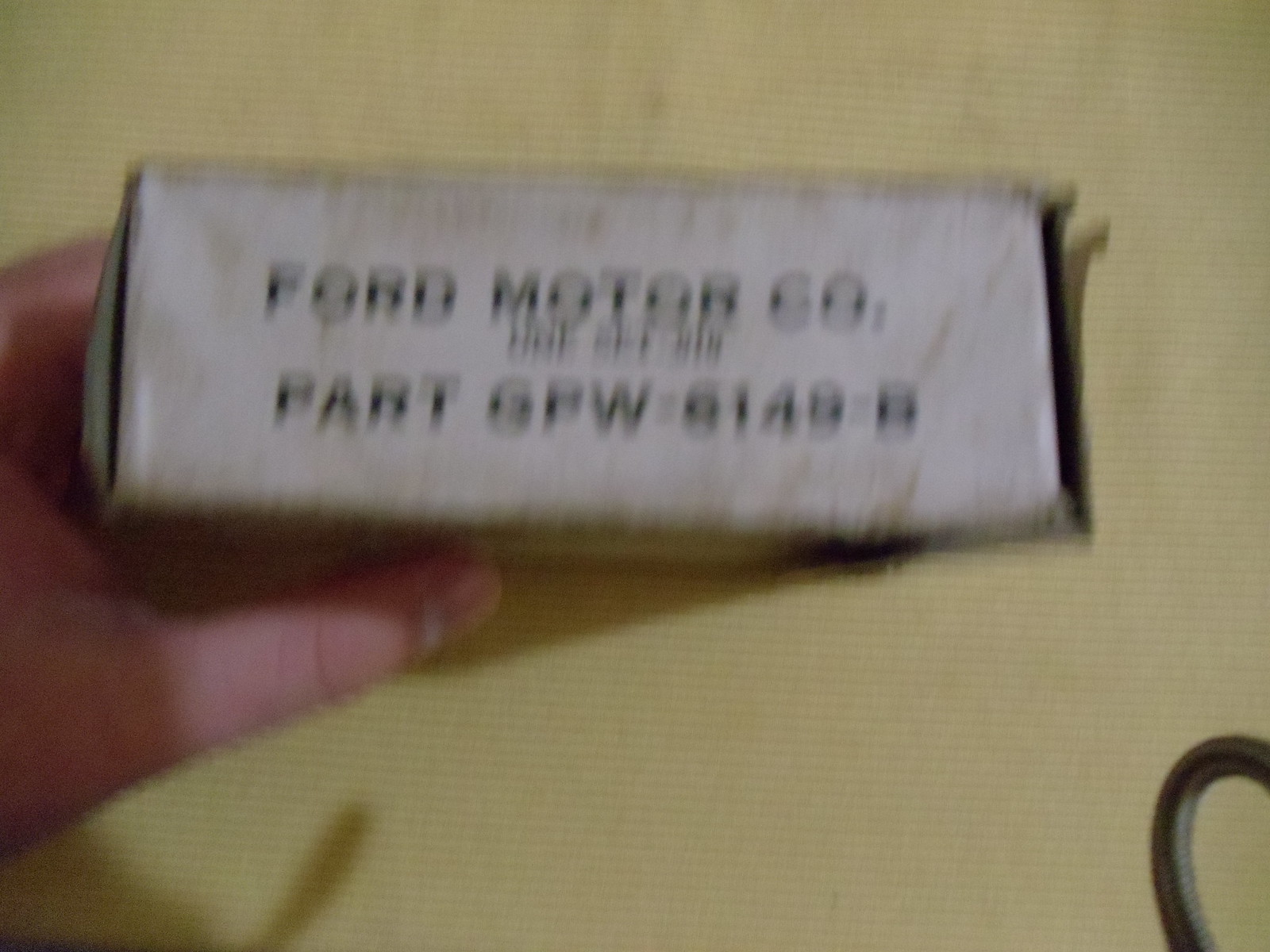This blurred image, captured from a head-mounted camera, shows the wearer's viewpoint. The background is a yellowish-brown fabric that fills the scene. Dominating the center of the photograph is a person's left hand, identifiable as Caucasian and slightly greasy, clutching a small, well-worn white box. The box bears black lettering that reads "Ford Motor Company" at the top, followed by the part number "GPW-6149-B." The hand is positioned from the left side of the image, with fingers wrapping around the back and a visible thumb holding the front. In the bottom right corner, the partial view of a metal loop or black curved object, perhaps resembling a handle or shoelace, is visible, adding an additional element to the frame.